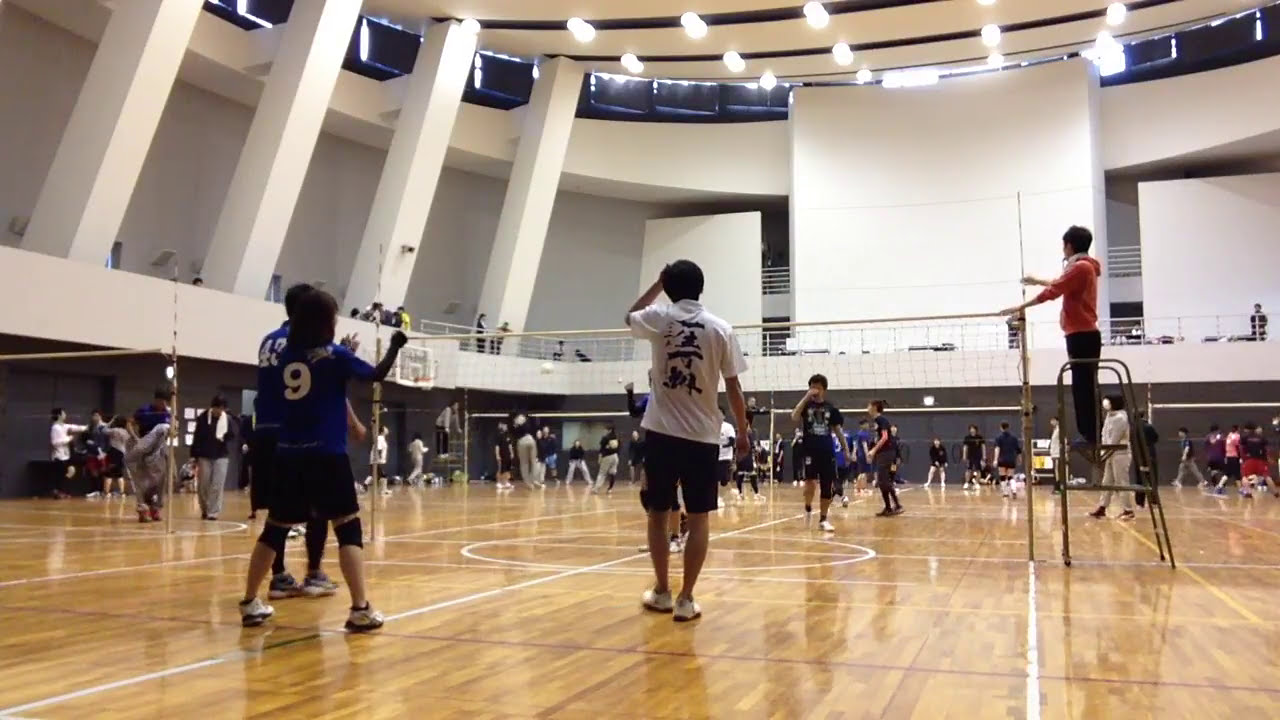Inside a brightly lit gymnasium, several volleyball tournaments are in progress, with multiple nets set up across the bustling floor. The gym hosts about 30 to 50 people, including numerous children, all appearing to be Asian, indicated by their dark hair and the Chinese and Korean letters on their jerseys, as well as their numbers. A high ceiling with white walls and abundant lighting illuminates the space, creating a lively atmosphere.

Dominating the foreground, a child in a distinctive blue uniform with the number 9 stands attentively with his hands in the air, while another boy in a white shirt, decorated in blue, accompanied by dark shorts and white sneakers, is positioned nearby. A young boy, possibly serving as the coach or referee, stands upon a ladder by the net, holding a whistle with determination.

In the background, a sea of children clad in vibrant uniforms continue their practice sessions, with some people watching from a higher level balcony connected by bridge-like stanchions. The gym floor is typical, featuring a brown and yellowish pattern, adding to the standard yet energetic vibe of the environment. Amidst the gameplay, some children are seen scratching their heads or faces, indicating a brief moment of reprieve during their engaging tournament.